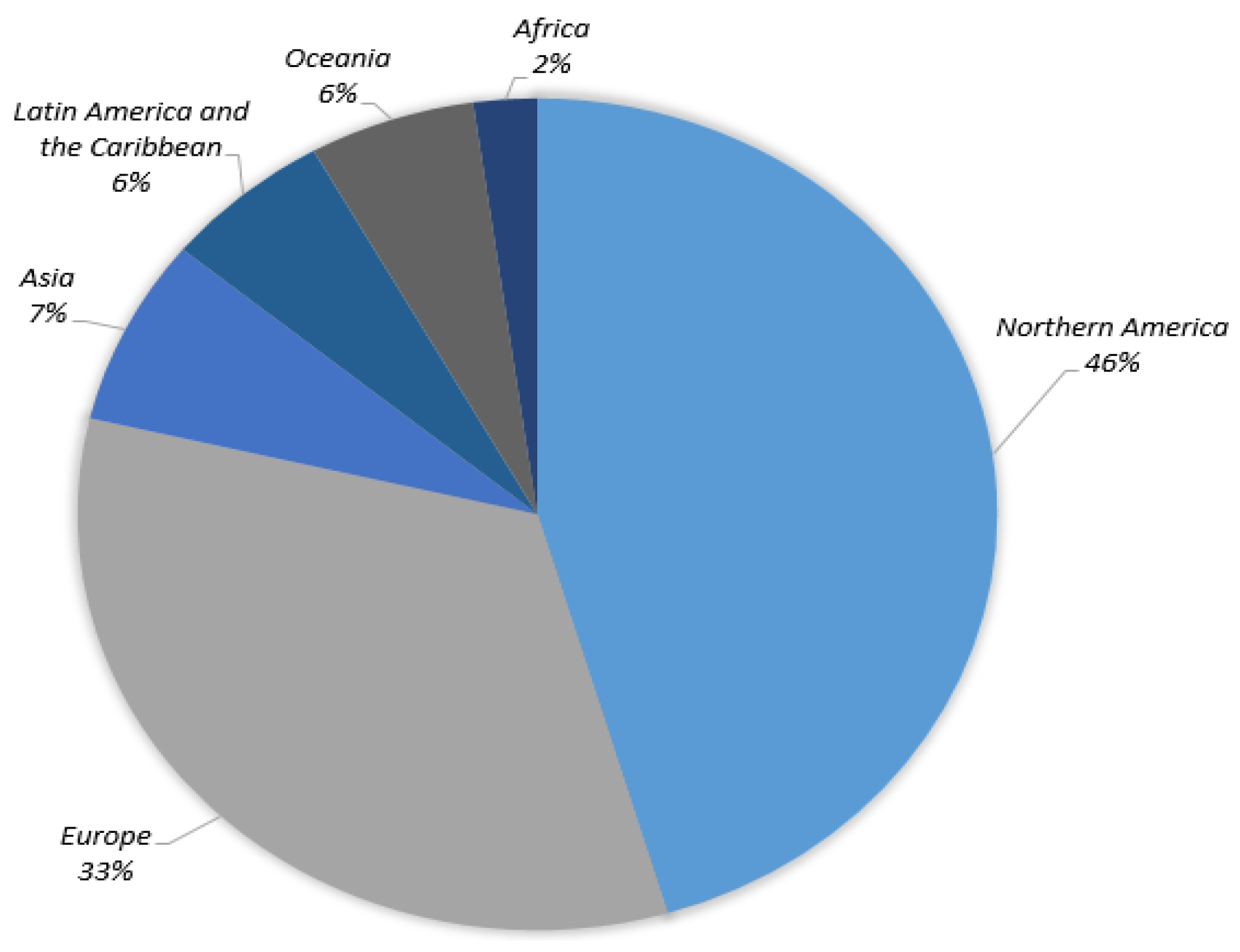The detailed pie chart displays the population distribution across various regions, each section distinctly color-coded. Occupying nearly half of the chart, North America is represented by a light blue segment, accounting for 46% of the total. Adjacent to North America, a very thin dark blue slice signifies Africa, making up 2%. Next, Oceania is shown in dark gray with 6%, while a similarly sized dark blue section represents Latin America and the Caribbean, also at 6%. Asia, in a standard blue shade, follows with 7%. Finally, Europe claims a substantial portion at the bottom of the chart, depicted in gray and representing 33%. The pie chart is set against a white background with black text labels positioned outside the circle, each connected to its respective segment by a line, ensuring clarity in data representation.